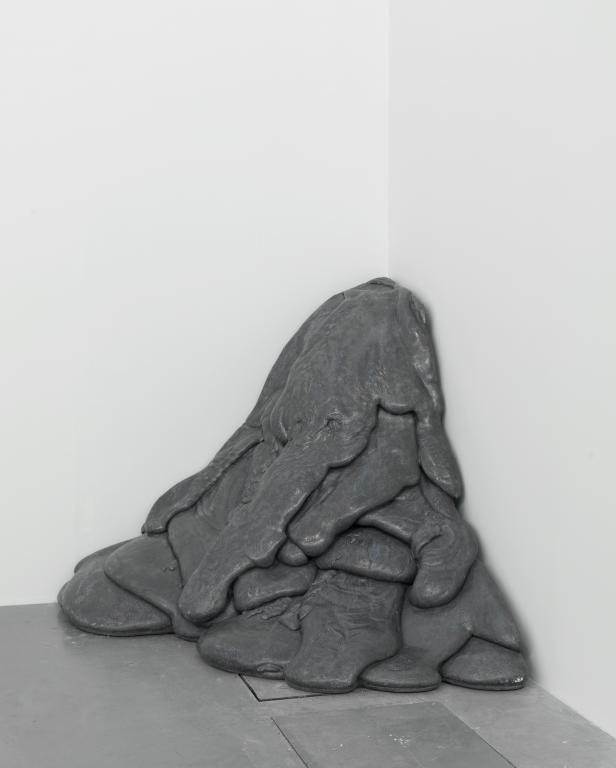This image depicts a striking sculpture set against the corner of a room with white walls and a gray concrete floor. The sculpture consists of layered, coal-black material resembling molten substances that have settled and cooled, forming undulating, oozing layers on the ground. Standing at about three feet in height, the texture of the sculpture is shiny and somewhat suggests a whimsical shape, reminiscent of a sitting elephant, complete with discernible wrinkles and an implied trunk. This dark gray, almost black creation starkly contrasts with the lighter, monochromatic surroundings, emphasizing its unique and imaginative form.